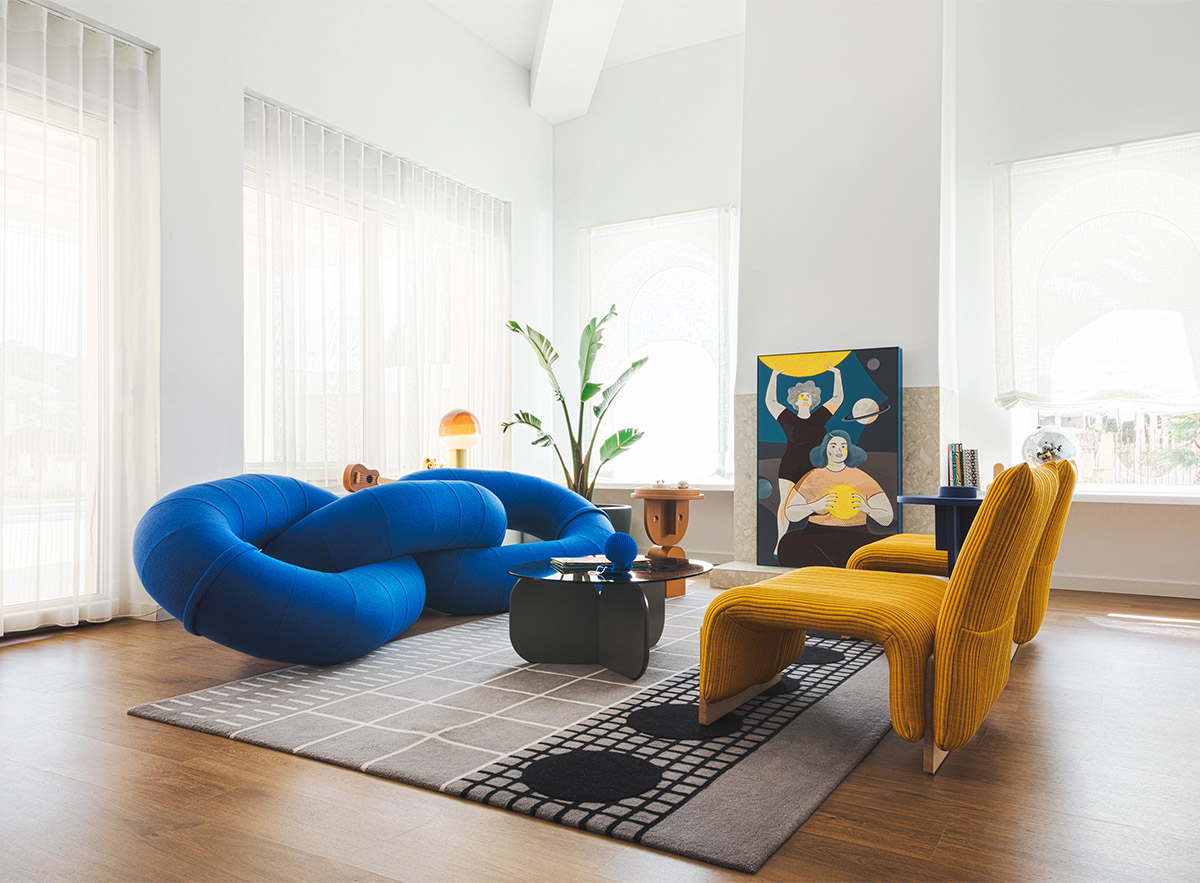The full-color square photograph depicts a modern indoor living room illuminated by natural light. The room features a dark brown hardwood floor, partially covered by a distinctive gray area rug adorned with black circles, white checkers, and patterned lines. The white walls and high ceilings add to the room's airy feel, complemented by several tall windows outfitted with translucent white drapes. 

The left side hosts striking full-size windows, while the center and right sides have standard picture windows. Dominating the center right wall is a notable painting of two women, with one holding a large yellow ball over her head and the other cradling a yellow ball at her chest, amidst various planets.

Furniture in the room includes two unusual yellow corduroy chairs placed on the right, described as "god awful ugly" and "strangely shaped." These chairs flank a small, sleek black coffee table and an adjacent blue round side table. On the left, there’s an unconventional blue couch, designed to resemble three interlinked chain oval loops, described as visually interesting but seemingly uncomfortable. Nearby, a brown wooden end table sits beside the couch. Additionally, a potted plant with large green leaves adds a touch of nature, enhancing the cozy yet avant-garde atmosphere of the living space.